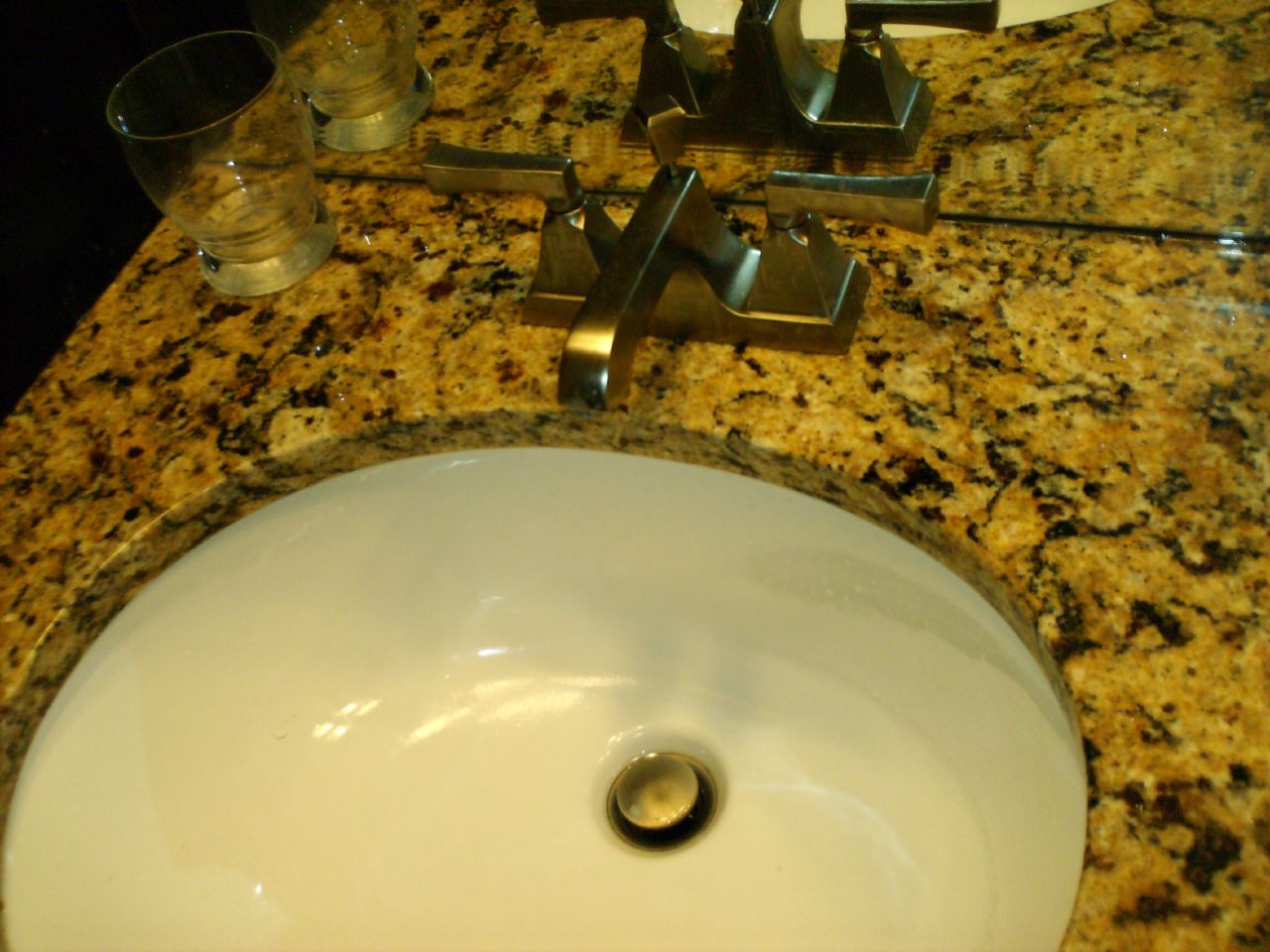The image showcases an elegant bathroom sink crafted from a marbled stone. The stone features a rich palette of beige tones that transition into brown, with subtle hints of very dark orange and tan woven into its glossy texture. The light softly reflects off the stone surface, highlighting its polished finish. The interior of the sink, under a lip of the same marbled material, is made of pristine white porcelain, presenting a classic look. A silver metal pop-up stopper sits at the bottom of the sink.

The sink is fitted with a silver metal faucet that includes two handles, one for hot and one for cold water. A central lever operates the pop-up stopper. On the left side of the marble counter sits an empty glass, the only item on the countertop. This glass is mirrored in the reflection behind the sink, where the faucet, marbled counter, and the hint of the sink bowl are also visible. The image captures the refined details and coordinated elements of this bathroom fixture, combining functionality with a touch of luxury.